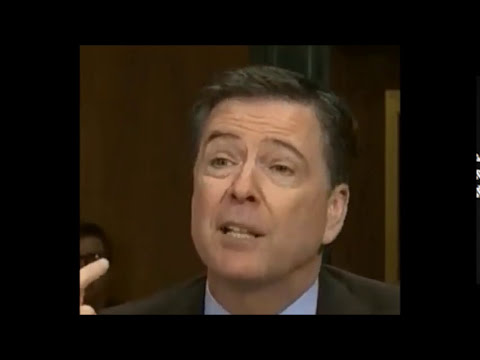The image appears to be a screenshot from a video, portraying a middle-aged white male at what seems to be a courtroom or formal setting. His short dark hair is parted to the side, and he is wearing a black coat over a white shirt. His forehead bears some noticeable stress marks. The man's mouth is slightly open as if he is speaking. Part of his shoulders and a bit of his index finger are visible. Behind him, the background consists of dark brown, likely wooden, walls. On the left side of the image, another person wearing glasses can be partially seen. The bottom left corner of the image shows fingers of a hand, cropped out. The entire image is encased in a thick black border, which is more pronounced on the sides than on the top and bottom. This scene is identified from one of Donald Trump's trials, featuring the former FBI director, James Comey.